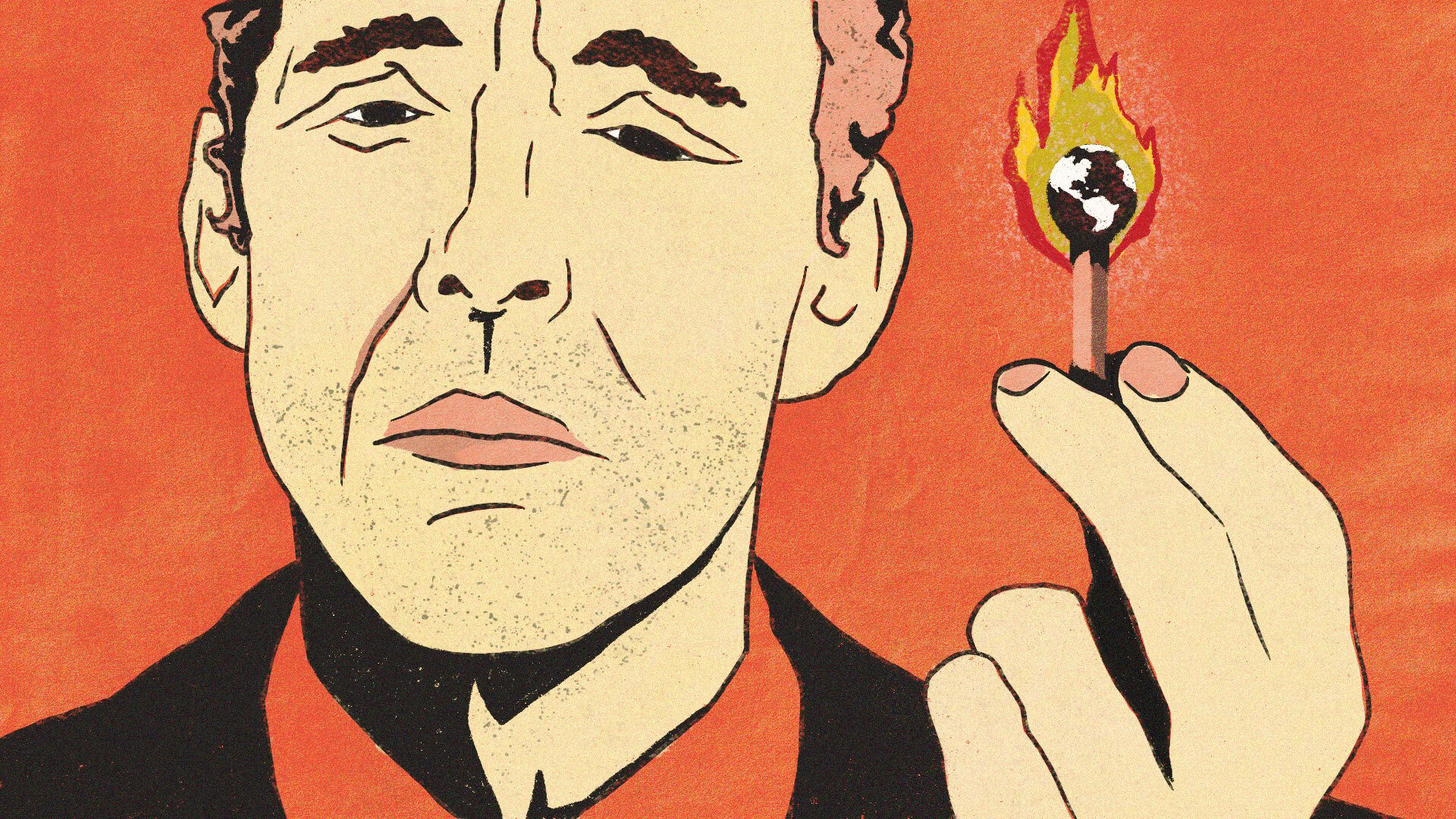In this detailed illustration, a cartoony, line-art depiction features a close-up of a man holding a lit matchstick in his hand, positioned to the right of his face. The matchstick is distinctively unique, with the match head fashioned into a globe, highlighting continents in white and brown, enveloped in a vivid yellow and red flame. The man’s appearance is notable; he has reddish-pink hair with black highlights, dark brown eyes, and bushy, dark eyebrows. His expression is pensive, almost mournful, complemented by a five o'clock shadow on his chin and mustache area. He wears a red collared shirt underneath a black jacket. The stark background is a bright orange-red, further emphasizing the scene’s intense and surreal commentary, likely on the theme of global warming and climate change. The illustration captures the man's visible despair over the burning earth, encapsulating a powerful and poignant message.